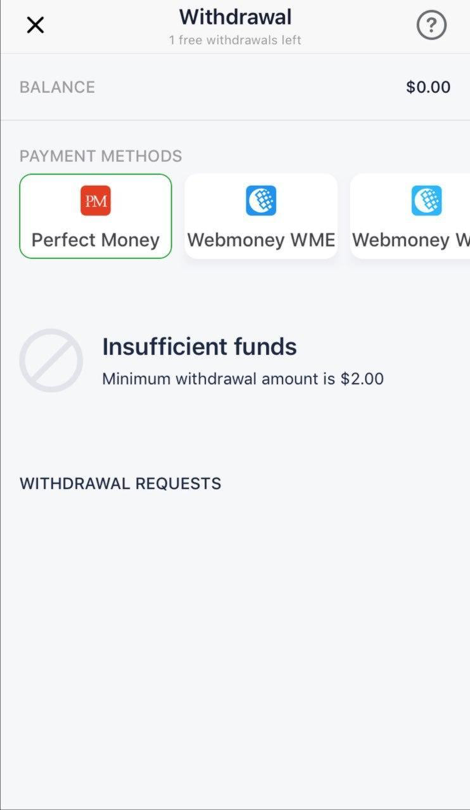This is a detailed screenshot from a financial banking app, showcasing the user's bank statement. The top of the image indicates "Withdrawals" with a note stating "three withdrawals left." The current account balance is prominently displayed as $0.00, indicating that there are no funds available in this account.

Highlighted in green is "Perfect Money," one of three displayed payment methods. Next to it is another payment method with a red logo. Additionally, there are two entries for "Web Money WME," although one is partially cut off and not entirely visible.

A large veto sign with the text "Insufficient Funds" appears below, emphasizing the account’s lack of money. The app specifies that the minimum withdrawal amount is $2.00. Further down, a section titled "Bonuses Withdrawal Request" is visible but currently shows no active or past requests.